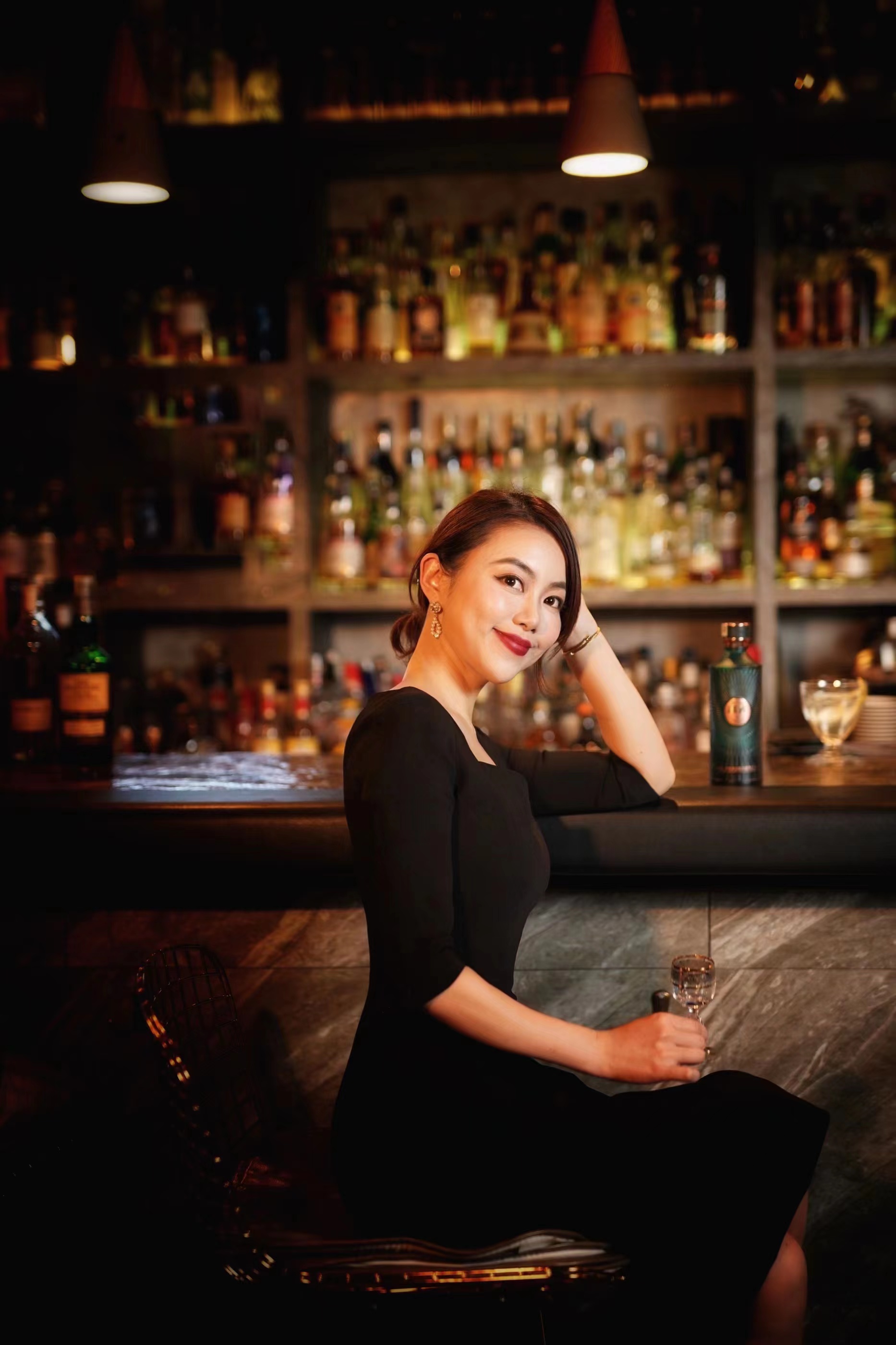In the image, a stunning young Asian woman is seated at a bar, elegantly dressed in a knee-length black dress with elbow-length sleeves. She is illuminated by pendant lighting that cascades down from the ceiling, giving the scene a warm glow. The setting is indoors, and the composition of the photograph suggests it was staged and modeled. 

The bar itself features a black marble façade with a darker bar top. She is sitting on a wooden chair with a small metal back, possibly cushioned, and the bar countertop is adorned with several bottles—at least three are placed to her left, one to her right accompanied by a large serving cup. Behind her, the back wall is lined with shelves displaying an array of liquor bottles and glasses, adding to the sophisticated ambiance of the scene. 

The woman, with her hair pulled back and adorned with earrings, exudes elegance. She has her left arm resting on the bar while holding a small glass beverage in her right hand, placed on her lap. She is smiling subtly towards the camera, her lips closed, and her demeanor portrays a poised and graceful profile as she glances slightly upwards and to the left, offering a side view of her charm.